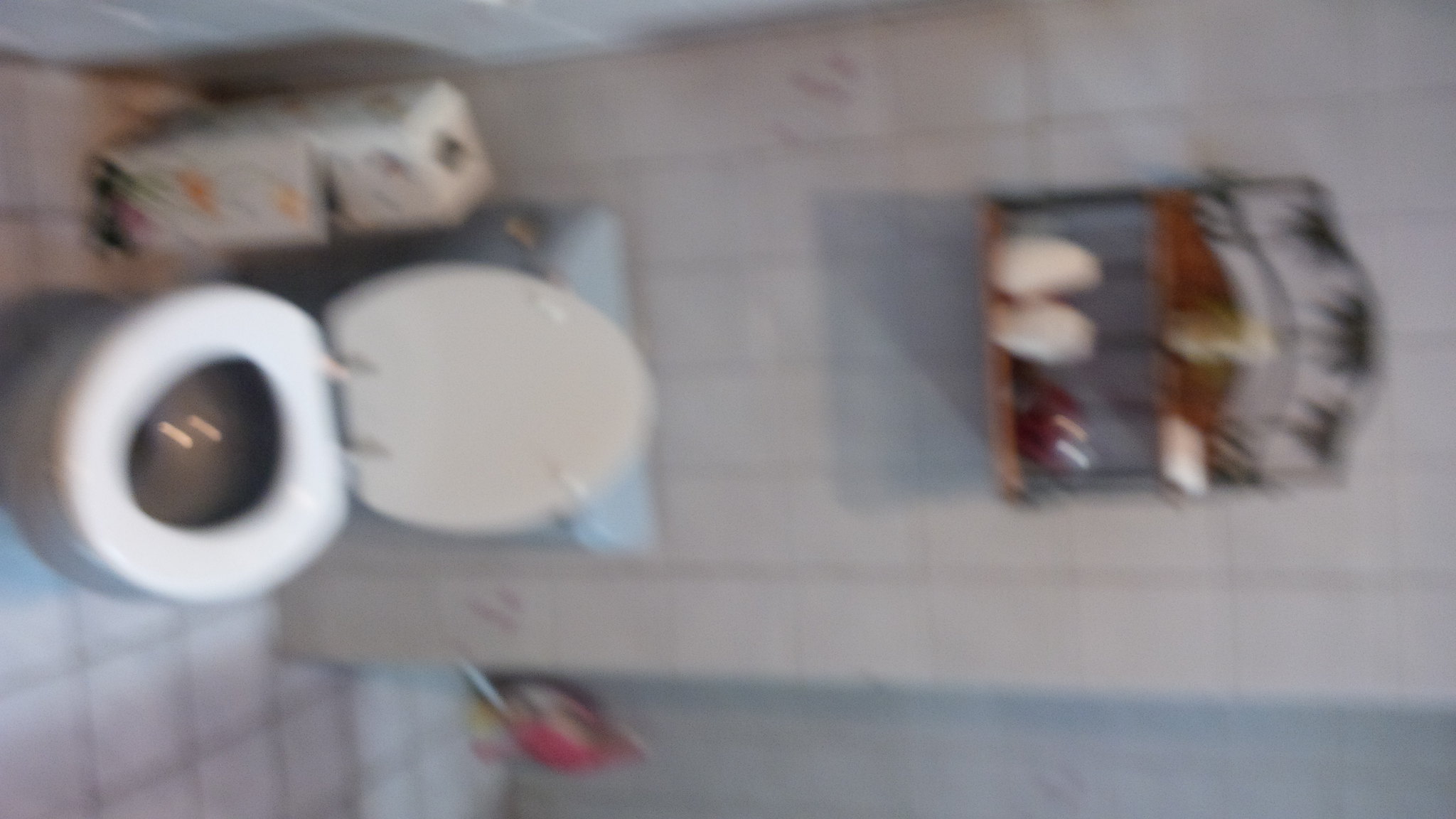The photograph is a blurry, sideways view of a public restroom stall. The main focus is a standard white toilet with an open lid, showing a light grayish bowl and a toilet tank with a light grayish-blue hue. The floor features white square tiles with brown grout, while the walls are lined with tan-colored tiles. Situated against the wall above the toilet is a hanging rack or basket, housing various toiletries including some large white containers and a few blue ones. Adjacent to the toilet, there is an object that appears to be a gray carry-on suitcase or a rectangular white box with labels, though the image blur makes it difficult to discern its exact nature.